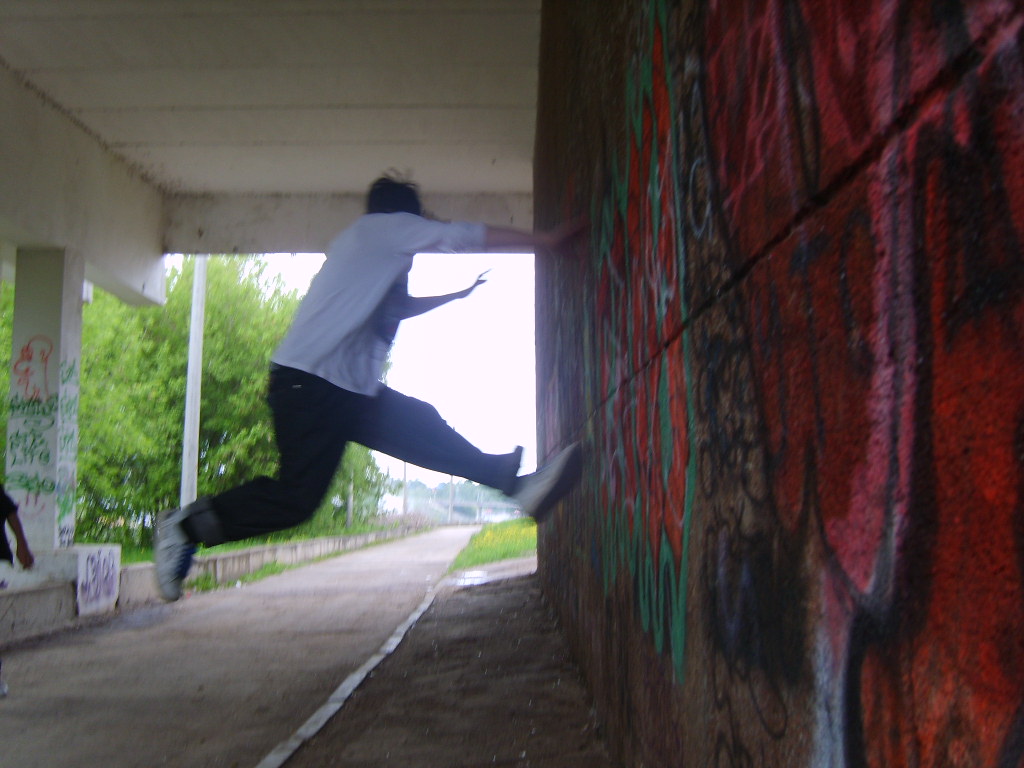This photograph captures an underpass footpath beneath a bridge, where the right-side wall is heavily adorned with graffiti in dark shades, dominated by reds, oranges, and greens. The surrounding atmosphere is dim, making it challenging to discern intricate details. The pathway, which might serve pedestrians or small vehicles, extends through the underpass. Central to the image is a young man, dressed in a white t-shirt, black pants, and white sneakers. He is leaping towards the graffitied wall with his left foot outstretched to make contact, his right foot trailing behind, and his right arm extended forward. Behind him, the path continues and is flanked by sparse trees and light poles in the background. The stark contrast between the vividly graffitied wall and the subdued colors of the rest of the scene accentuates the dynamic motion of his jump.